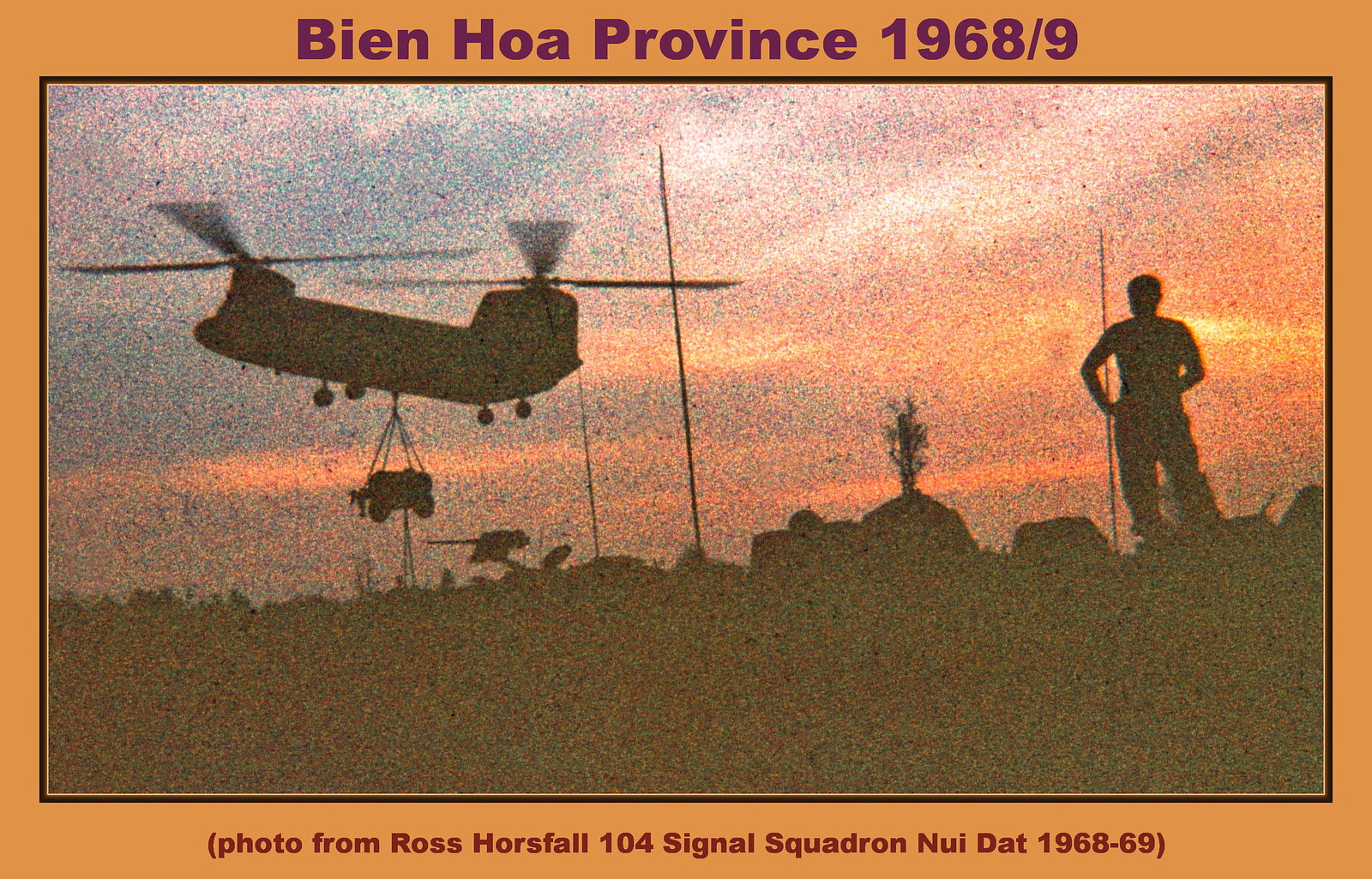The dusk photograph, bordered in orange with purple text, showcases a powerful scene from the Vietnam War. The text at the top of the frame reads "Bien Hoa Province, 1968-1969," while the bottom credits "photo from Ross Horsfell, 104 Signal Squadron, Nui Dat, 1968-1969." The image captures the silhouette of a dual-rotor helicopter suspending a load beneath it, casting stark shadows against a pastel-hued sky in shades of orange, pink, red, and bluish tones that blend together artistically. A soldier stands to the right, observing the aircraft in the fading light. The foreground details, including plants, rocks, and poles, are also silhouetted, contributing to the photograph's dramatic and evocative composition.